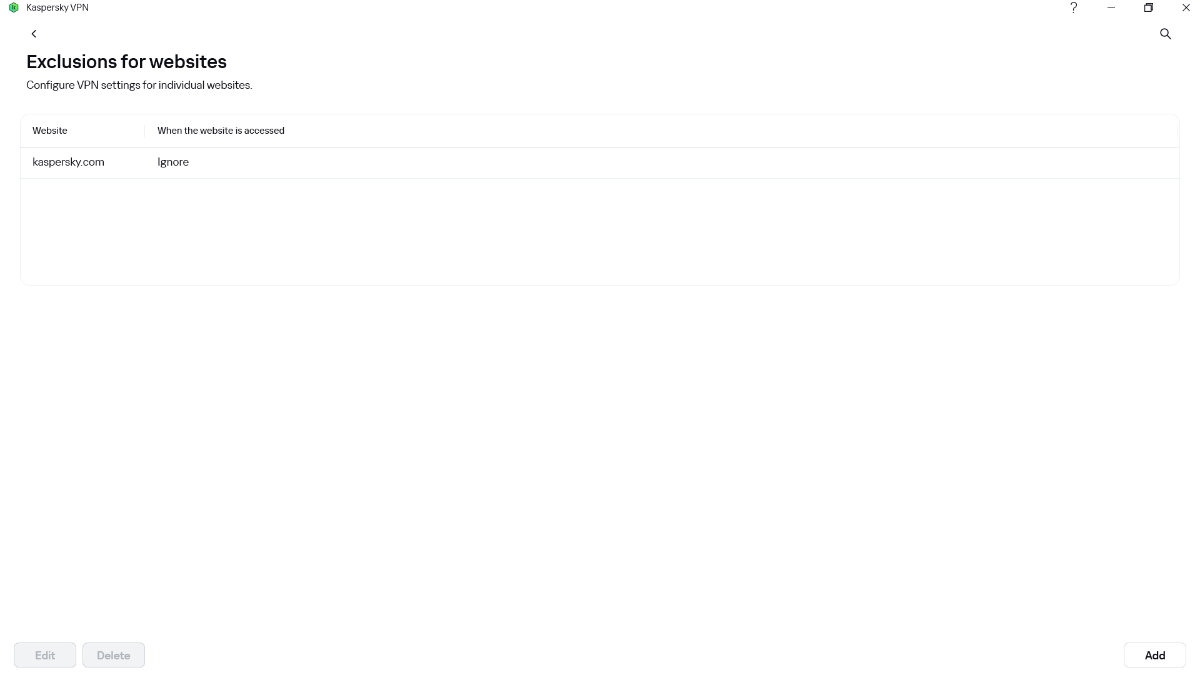Caption: 

The image depicts the Kaspersky VPN application on a Windows system. In the upper left-hand corner, the title "Kaspersky VPN" is prominently displayed, accompanied by the standard Windows interface buttons for minimize, close, and maximize. Additionally, there are question mark and search magnifying glass icons in this section.

Under the main title, there's a bold heading that reads "Exclusions for websites," which indicates the section where users can configure VPN settings for specific websites. Following this, the text details the current exclusion, which is "Kaspersky.com," set to be ignored by the VPN.

At the bottom left of the screen, there are "Edit" and "Delete" buttons, though they are currently grayed out and inactive. In the bottom right corner, there is an "Add" button, distinct with a white background, black text, and a light gray border.

End Caption: "Thanks for watching. I hope you found this helpful. If you did, please like and subscribe, and I'll see you in the next video."